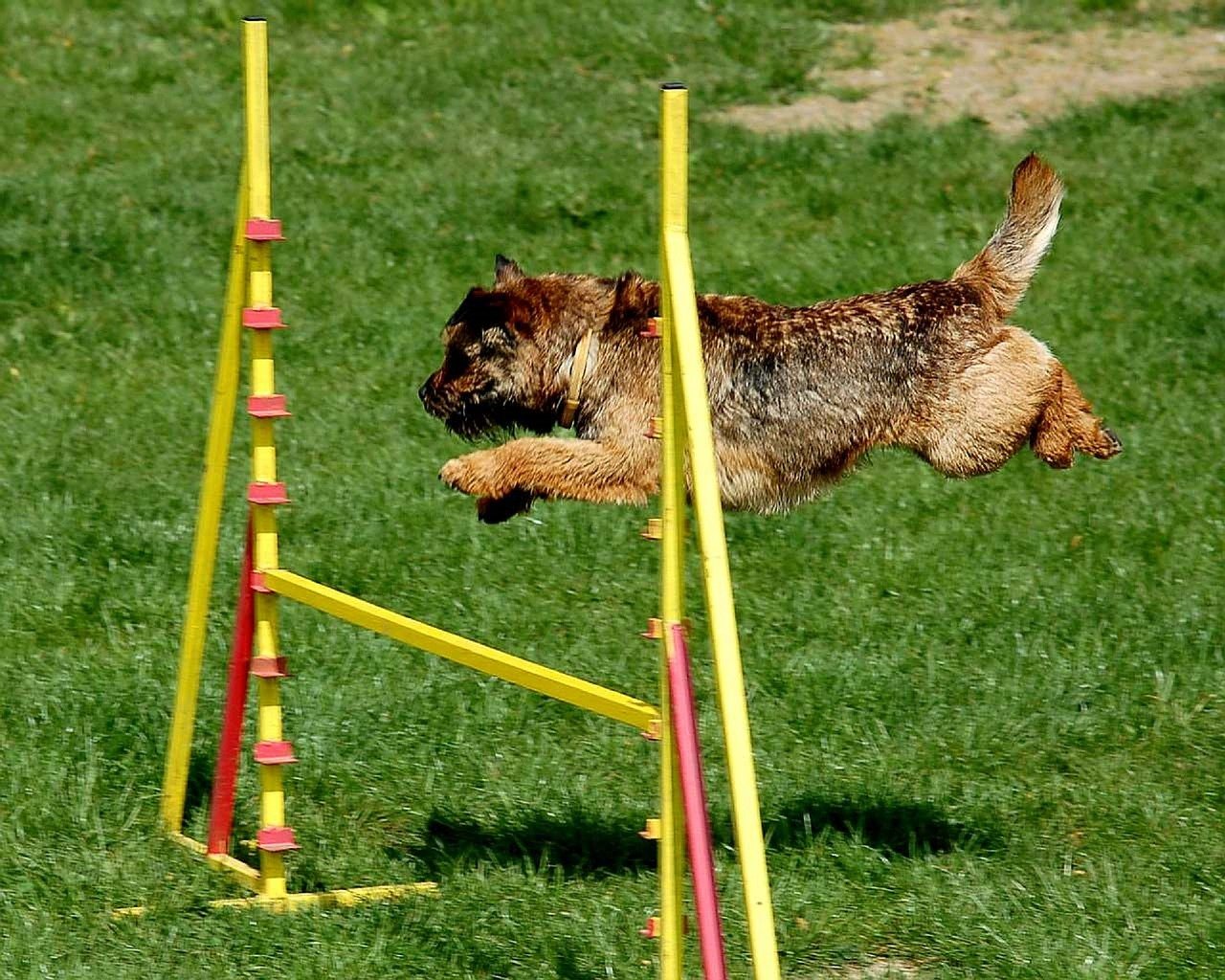A lively brown dog, with mottled fur and a slightly shaggy appearance, is captured mid-leap as it soars over a red and yellow hurdle in what appears to be an agility trial. The dog's coat features a variety of brown shades, with darker hues around its head, midsection, and the base of its tail, and lighter patches towards its hind legs and front legs. The dog's light brown collar is visible as it fully extends its front legs forward and back legs behind, demonstrating impressive speed and agility by jumping significantly higher than the one-foot height of the hurdle. The yellow hurdle comprises two yellow poles with adjustable red tracks, set against a background of patchy dark green grass, which transitions into a clearing with light brown dirt. The daytime setting illuminates the scene, highlighting the dog's athletic prowess and the vibrant colors of the hurdle.